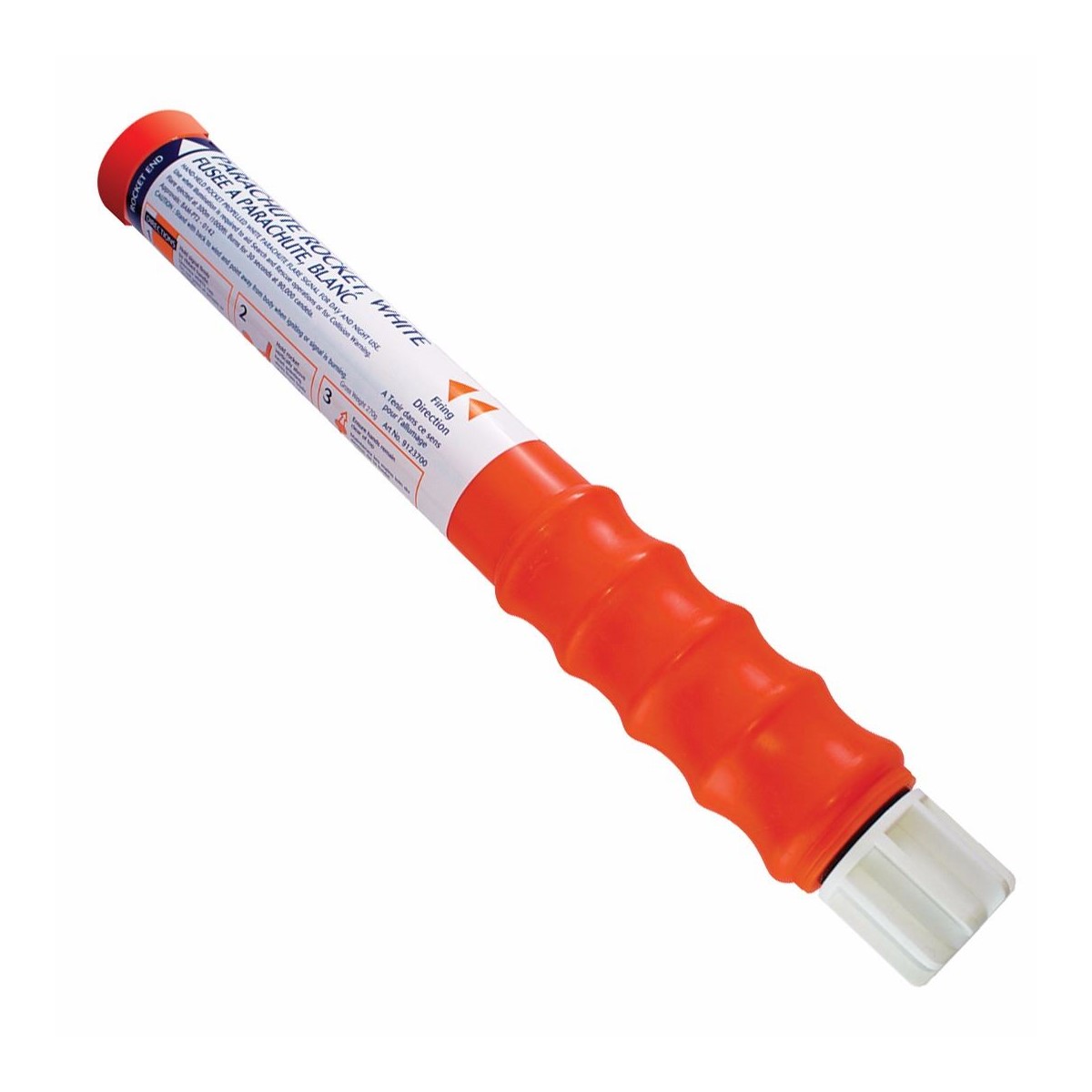The image depicts a cylindrical product resembling a pipe or a large EpiPen, with a predominantly orange body. One end of the cylinder features a white, knob-like cap, which is pointing towards the bottom right. The product also has a ribbed or knurled grip area, suggesting it is designed for easy handling. This grip area is also orange. A wide, white label with black text is wrapped around the middle of the product, with part of the text in capital letters reading "PARACHUTE ROCKET WHITE FUSE A PARACHUTE BLANK," followed by additional smaller text. The label might contain usage instructions or other relevant information. The background of the image is entirely white, providing a clear contrast to the orange and white product, making it the focal point of the photograph.